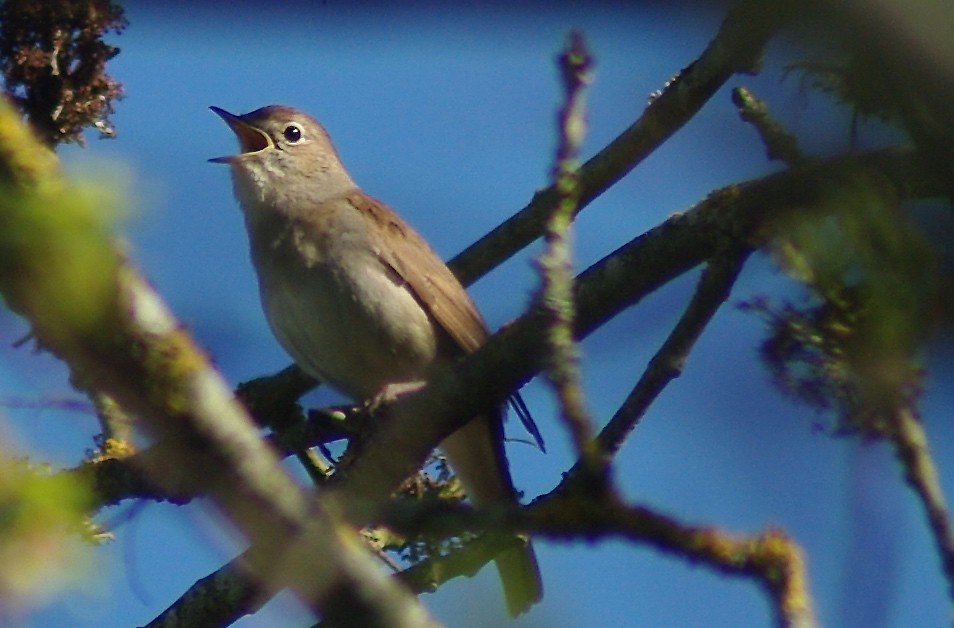This image captures a small brown bird with a grayish-white belly perched on a tree branch. Its beak is open mid-call, suggesting it's making a sound or calling out into the distance. The bird features black circular eyes and a long tail. It's positioned slightly to the left within the frame, looking towards the top left of the picture. The surrounding branches, some of which are blurred, bear a mix of green and brown leaves. A clear, bright blue sky with no clouds serves as the backdrop, enhancing the vividness of the scene. The photograph focuses tightly on the bird, emphasizing its details and the natural setting.